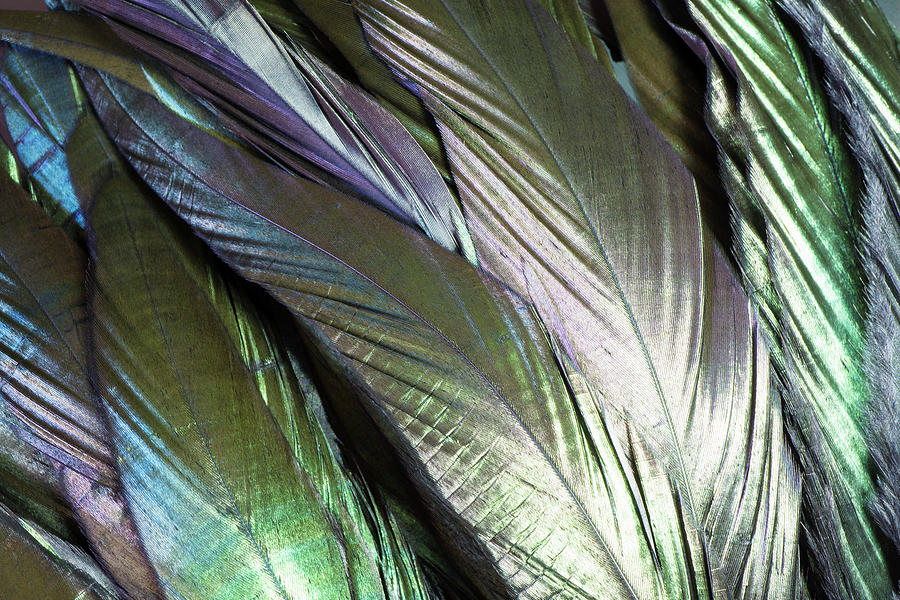This is a close-up photograph showcasing a striking array of large, tropical-looking leaves that possess an iridescent, spray-painted appearance. The leaves, overlapping and laid together, display a dazzling spectrum of colors as light reflects off their surfaces. Predominantly, these leaves appear in shades of metallic green, purplish, pink, and yellow, creating an impression of silvery feathers, possibly from a vibrant bird like a peacock, but more likely artificial due to their vivid, reflective sheen. Positioned within a rectangular frame, the leaves cascade from top to bottom, with their colors shifting from green to purple to black and blue, before transitioning to a light purple and culminating in a mesmerizing blend of green, white, and purple on the far right. The brilliance of the sunlight captures the iridescence perfectly, making the composition a captivating study in color and texture.